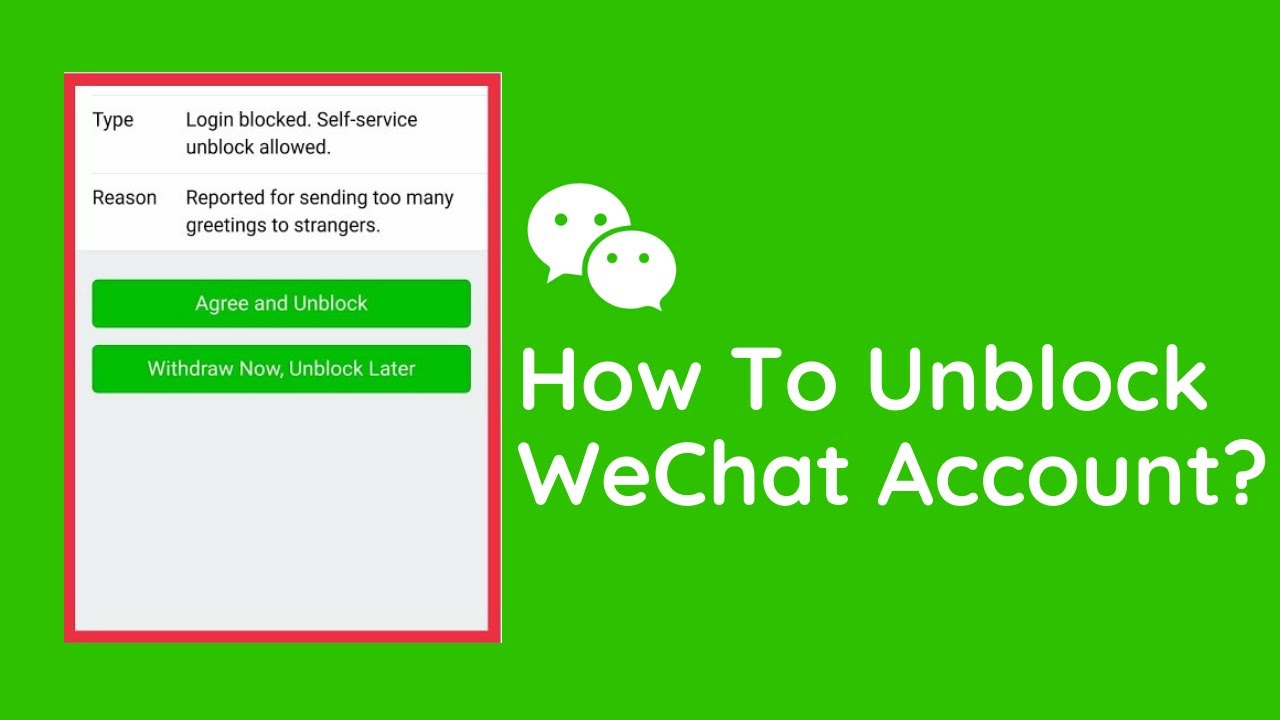Here is a cleaned-up and detailed caption for the image:

---

Screenshot of an instructional page titled "How to Unblock WeChat Account?" The screenshot features a prominent bright kelly green rectangle as its background. In the center of the green rectangle is a white, red-bordered rectangle situated towards the left side of the image. 

Inside this white rectangle, the instruction begins with "Type" in black font, followed by "Login Block" and "Self-Service Unblock Allowed" written in red font. Below that, "Reason" is in black font, with the explanation, "Reported for sending too many greetings to strangers," also in red font.

Towards the bottom of the white rectangle are two green buttons with white text. The first button reads "Agree and Unblock," while the second button reads "Withdraw Now, Unblock Later." At the top of the green background, positioned above the text, are two white quotation bubbles.

---

With these details, the caption provides an in-depth description of the content and layout of the screenshot.